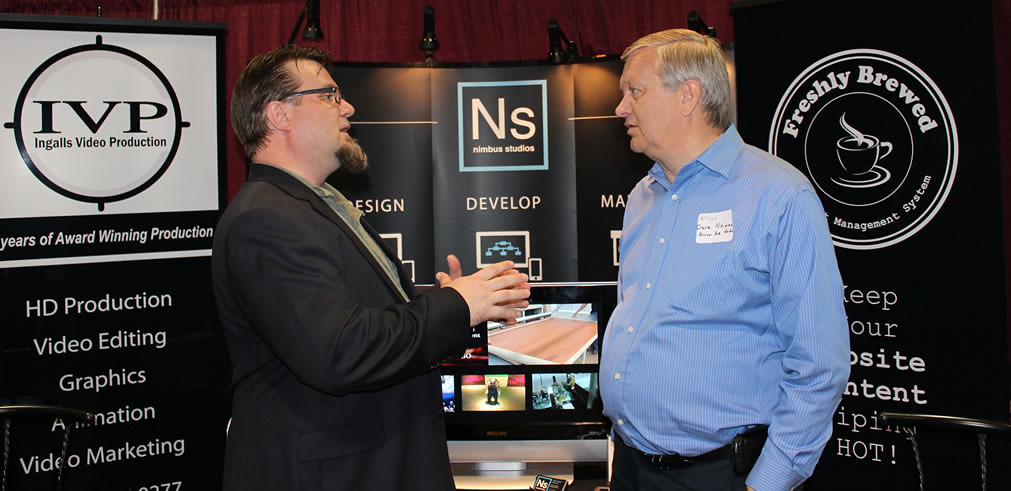In this image, two men are conversing at what appears to be a conference or trade show. The man on the left is wearing a dark suit jacket over a tan button-down shirt. He has brown hair, light skin, glasses, and a well-groomed beard, and is clasping his hands in front of him as he talks. The man on the right, slightly older with gray hair, is dressed in a blue long-sleeve shirt and black pants, with a white name tag pinned to his chest. He has a slight belly and is clean-shaven. Both men appear to be in their late 40s or early 50s.

They are standing in front of a multi-panel display with a dominant black background and white text. On the left side, the display features the logo "IVP" and the name "Ingalls Video Production" encircled. Underneath, it touts "Years of award-winning production" and lists services such as "HD Production, Video Editing, Graphics, Animation, and Video Marketing." To the right, there is a display board for "Nimbus Studios (NS)," identified by a blue box with "NS" and the word "Develop" beneath it, along with some small, hard-to-see icons and images.

In the upper right corner of the image, another part of the display highlights a circle with a coffee cup image and the words "Freshly Brewed." Surrounding this, the circle includes phrases like "Management System" and "Keep our website content piping hot." The combination of these detailed displays and the men's engaged conversation strongly suggests the setting is professional and related to video production and digital content.